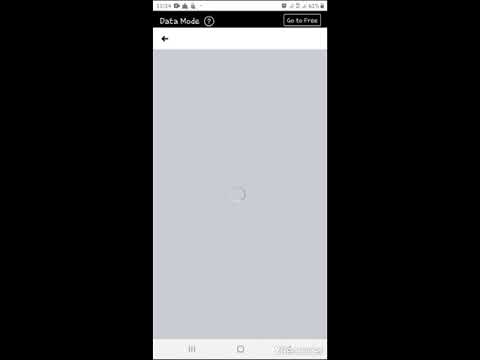The image displays a loading screen from the Facebook app. At the top, there's a black header with white text. On the top left, the header reads "Data Mode" followed by a white question mark inside a white circle. Adjacent to this, on the right side, it says "Go to Free" with an icon of a white triangle beside it. 

Centered in the middle of the screen is a loading circle, colored in a silver-grey hue against a grey background. On the top left, just below the header, there's a back button, depicted as a left-pointing arrow in black, which navigates to the previous menu when pressed.

The bottom of the screen showcases the standard smartphone navigation buttons: minimize, home, and recent apps. The left and right sides of the page are black, while the entirety of the content is centered and oriented in portrait mode.